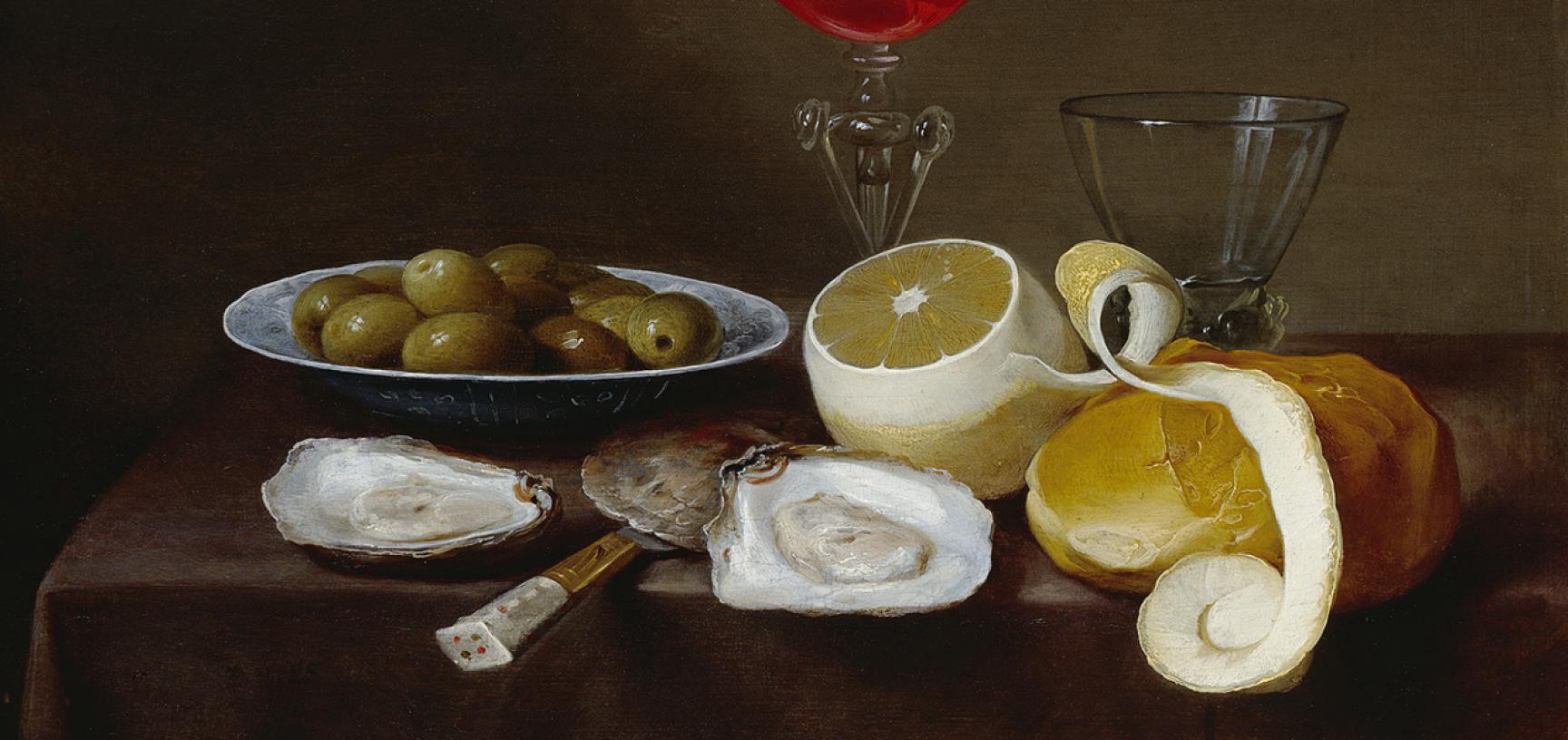This highly stylized photograph showcases an artfully arranged assortment of food items on what appears to be a vintage, dark maroon tablecloth-draped wooden box or footlocker, set against a rustic, dark gray or olive-brown wooden wall. The lighting casts shadows that add to the moody and dramatic atmosphere of the scene. At the center and spreading to the right, a peeled grapefruit with sections visible at the top has its peel cascading in a spiral over the scene, draping elegantly over a partially sliced loaf of light beige bread positioned at the rightmost corner. To the left, a white plate holds a generous pile of approximately 12 to 15 large green pimento-stuffed olives. In front of the plate, two shucked oyster shells with white interiors nestle beneath a slender, tall glass bowl. A V-shaped clear glass bottle with a prominent red cork and an empty clear water glass are placed behind these items. The interplay of the textures from the peeled fruit to the rough wood and smooth glass creates a rich, tactile composition, all arranged meticulously on the elegantly draped tablecloth.